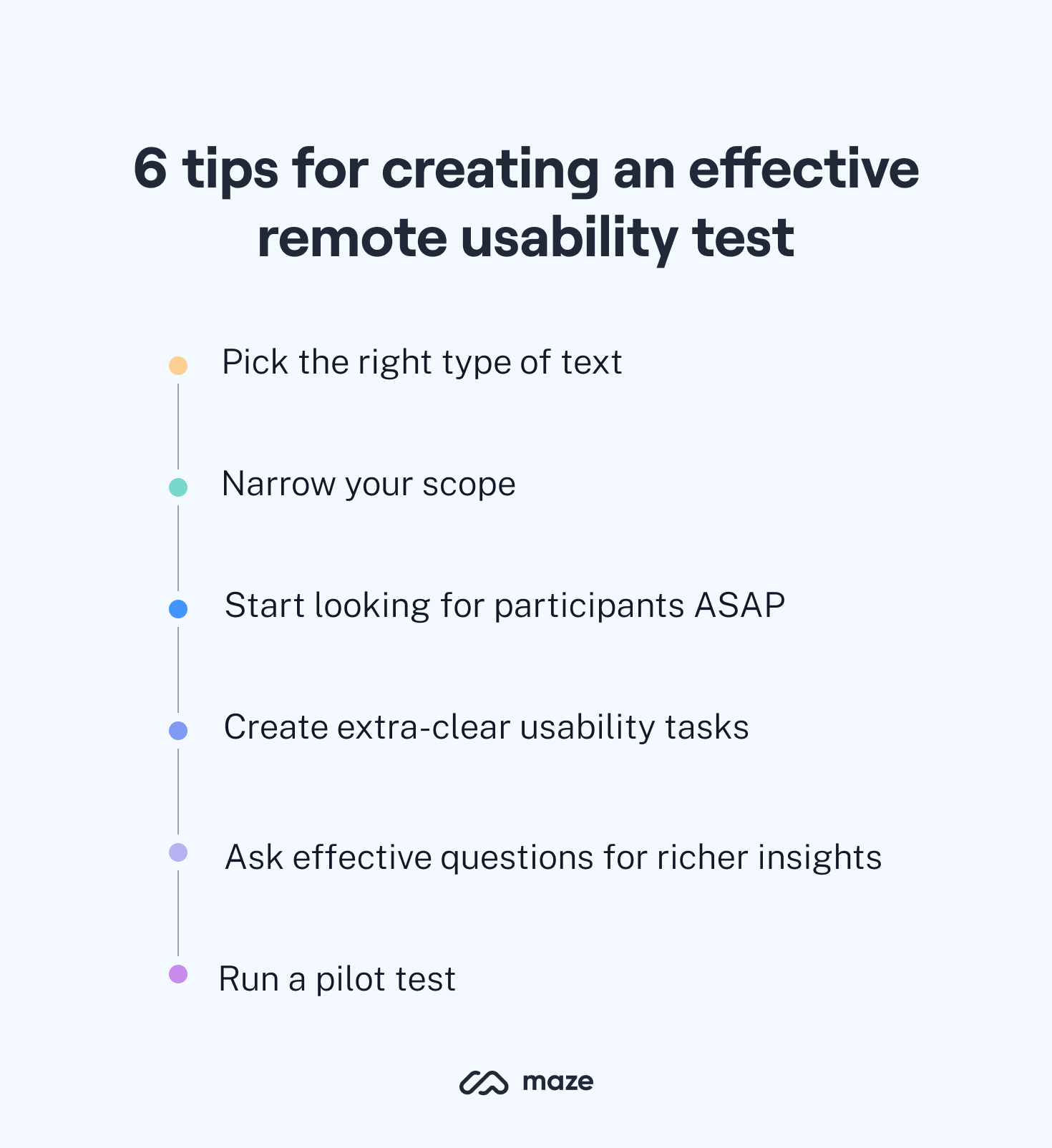The image is a detailed digital poster with a blue background, likely from an app or website, titled "Six Tips for Creating an Effective Remote Usability Test" in big, bold, black font at the top. Below the title, there are six bullet points, each accompanied by different colored dots and connected by a horizontal line, forming a visual guide. The bullet points are as follows: 

1. "Pick the right type of text" marked with an orange dot.
2. "Narrow your scope" marked with a greenish-turquoise dot.
3. "Start looking for participants ASAP" marked with a blue dot.
4. "Create extra clear usability tasks" marked with another blue dot.
5. "Ask effective questions for richer insights" marked with a gray dot.
6. "Run a pilot test" marked with a purple dot.

At the bottom center of the poster, there is a logo with the name "Maze" displayed. The poster serves as a structured, colorful guide to conducting remote usability tests effectively.